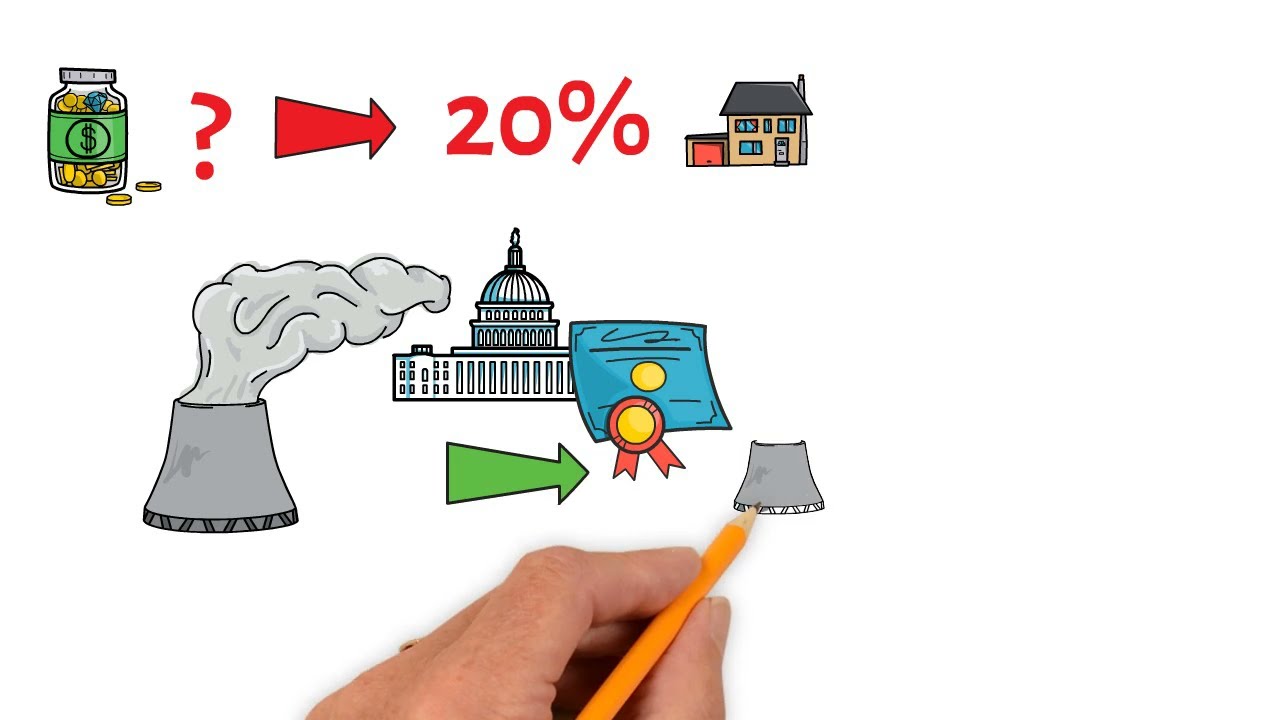The image features a white background and appears to be a scene from an explainer video. Dominating the lower portion is a lifelike left hand holding a yellow pencil, actively drawing. The hand is sketching a gray cement tower resembling a power plant silo emitting smoke. Another finished silo, also letting off steam, is seen to the left. To the right of the partially drawn silo, there is a green arrow pointing towards it. 

Above this section, the upper part of the image displays a series of clipart objects arranged horizontally. From left to right, the sequence begins with a glass jar filled with coins, labeled with a green dollar bill. This is followed by a red question mark, then a red arrow pointing right with the text "20%." Lastly, a brown house with a brown roof and red garage concludes the top row of drawings. Below these, near the hand, illustrations include the White House or a Congress-like building, a certificate or diploma, and the green arrow that points towards the ongoing drawing of the silo. The entire composition, except for the realistic hand and pencil, consists of cartoon-style visuals.